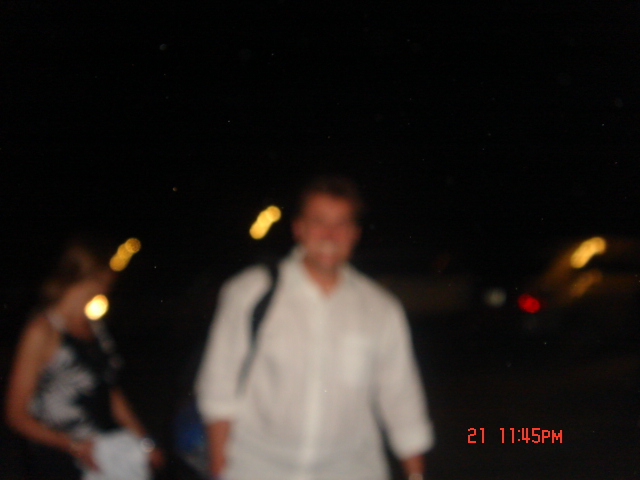This is a very blurry nighttime color photograph of two people with a timestamp "21-11:45 p.m." in bright red in the bottom right corner. In the center is a man with tan skin, wearing a long-sleeve white cotton dress shirt rolled up to the elbows, and a black or blue backpack over his right shoulder. He has short brown hair and appears to be smiling slightly, but the clarity of his facial features is hindered by the blurriness. To the left, there is a woman with blonde hair pulled back into a bun, wearing a sleeveless black and white patterned dress. She holds a white sweater in her hand and is looking behind her, adding to the sense of motion. Behind them, the background is punctuated with various series of bright lights: three to the right of the man's ear, three more on the far right of the photograph, and a series of lights above the woman's head. The lighting adds to the photo's hazy, dreamlike quality.